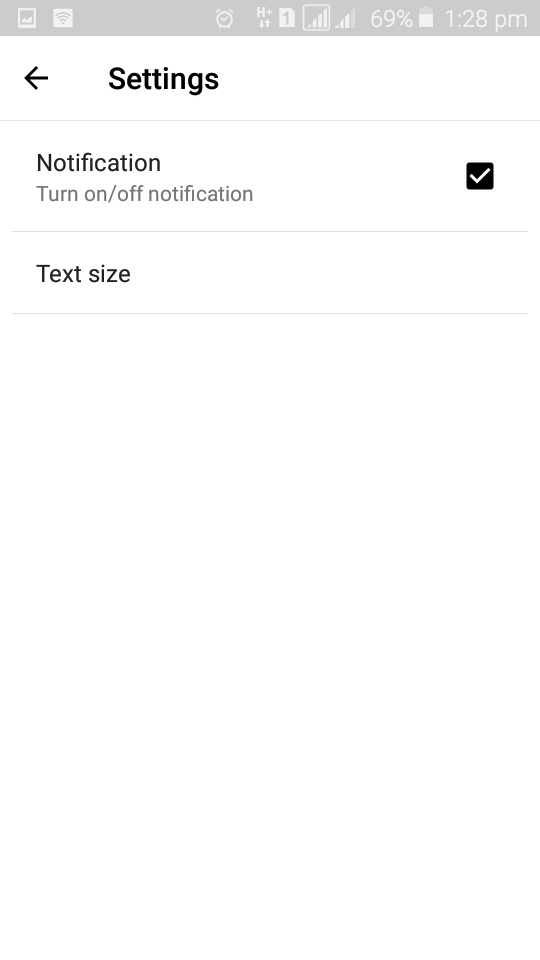This rectangular image, approximately one and a half times wider than it is tall, appears to be a screenshot of a settings page, likely from an application or a device. The image is framed by a light gray border on the top, with the main portion of the page being white and borderless.

At the top in the gray border, there are two white icons on the upper left. The first one looks like a box with bar graphs or line graphs inside, and the second resembles a Wi-Fi signal indicator, except it has a white background and gray inside. To the right of these icons, stretching left of the center due to the quantity, are six more icons:

1. An alarm clock icon
2. The text "H+" with several small symbols beneath it
3. A white rectangular portrait box with a snipped upper right corner
4. A white-outlined box with gray insides and a white ascending bar graph forming a right triangle
5. A similar ascending bar graph without a surrounding box, where the first three bars are white and the last is light gray, next to "69%"
6. A clipboard icon followed by "1,28" and "PM" in lowercase

In the bulk of the image, the top left corner features a squat black arrow pointing left, with the word "SETTINGS" in bold, black, initial caps to its right. A thin gray underline spans the length of the image below this header.

Two main sections follow beneath this underline, both slightly indented. The first section, labeled "NOTIFICATION," has a subtext in a smaller font stating "TURN ON/OFF NOTIFICATION." To the right of this text is a black box with a white checkmark. Another gray line separates this from the next section, which is labeled "TEXT SIZE" in capital T and lowercase for the rest. There is also an underline beneath. 

Both sections are left-justified and indented slightly more than the left-pointing arrow but less than the word "SETTINGS." This detailed description encapsulates the structured design and specific elements of this settings page.